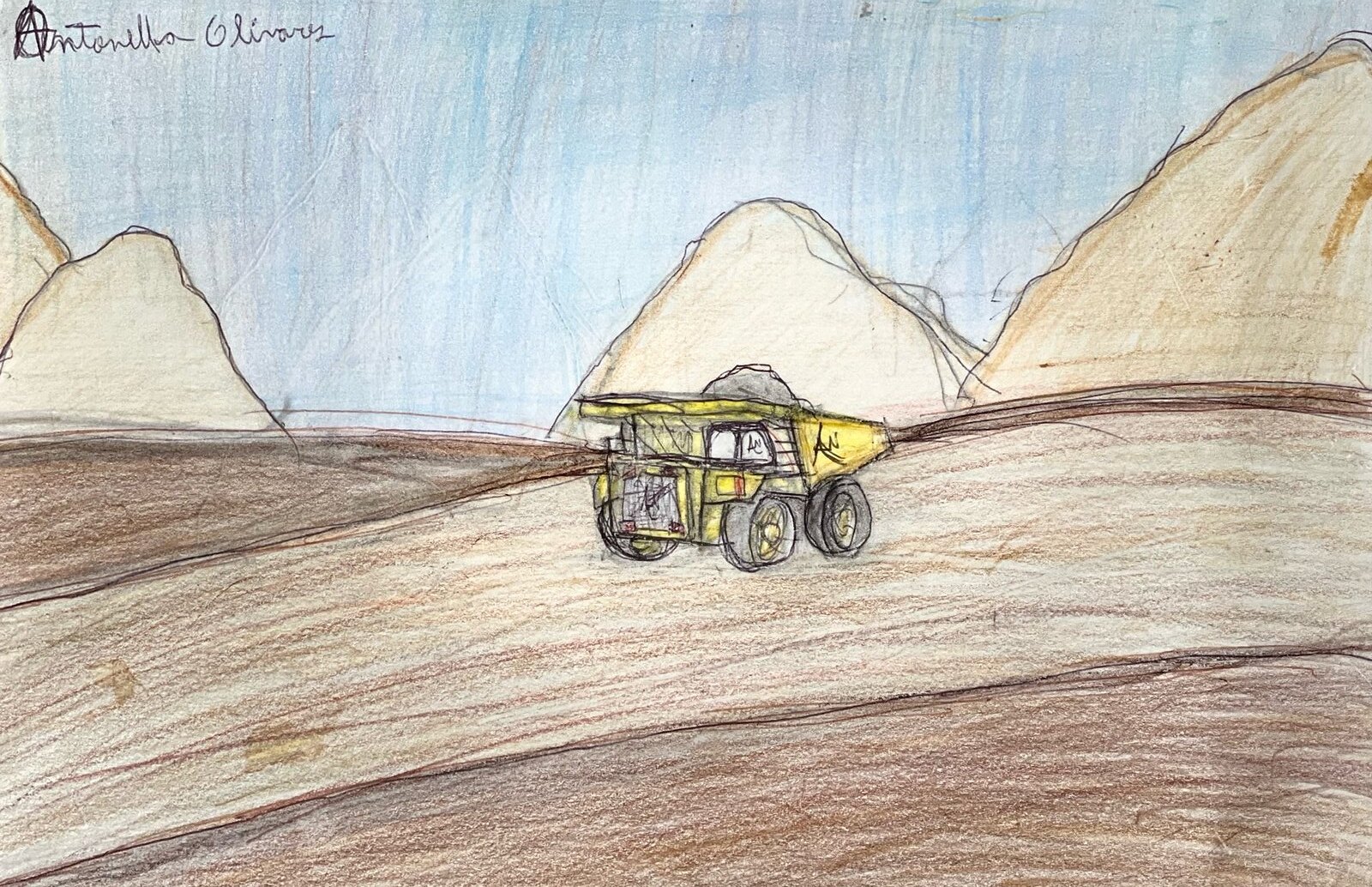This hand-drawn illustration, seemingly the work of a child, prominently features a yellow dump truck with distinctive black wheels and yellow headlights. The truck, positioned centrally, carries a load of gray material, possibly sand or gravel, in its bed. Crafted with colored pencils, the scene is set against a backdrop of light brown mountains and brown hills with darker edges, sketched with quick, jagged strokes. The sky above is filled with light blue pencil shading. In the top left corner of the image, the artist's signature, “Antonella Olivares,” written in black ink in a cursive style, stands out, with a distinctive "A" reminiscent of the Anarchy symbol encircled. The illustration exudes a playful, chaotic charm typical of youthful artistry.